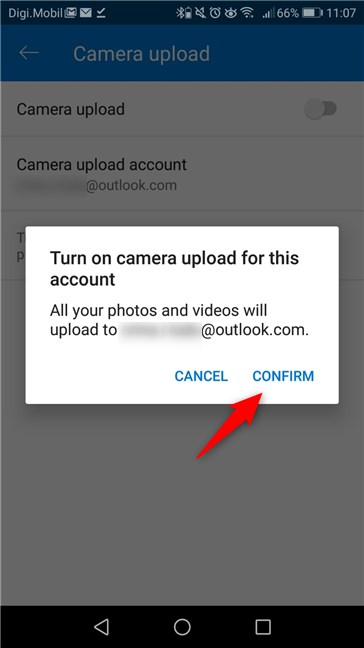The image is a screenshot from a mobile phone. The background starts with a blue gradient at the top, transitioning to white, with an overall gray overcast due to the brightness of a central white pop-up box, casting a dim effect on the rest of the screen.

**Pop-up Box:**
- **Title:** "Turn on camera upload for this account" in black text.
- **Description:** "All your photos and videos will upload to [email protected]", with the email address partially blurred for privacy.
- **Buttons:** Two blue options at the bottom right - "Cancel" on the left and "Confirm" on the right, with a red arrow pointing to "Confirm".

**Top Bar:**
- **Content:**
  - On the left: "DigiMobile" in blue.
  - At the center: a white box with a blue "M".
  - To the right: a series of white icons including an envelope, a check mark underlined, the Bluetooth symbol, a battery, a muted horn, an alarm clock, and an eye. 
  - Further right: Wi-Fi signal strength bars, phone signal strength bars, "66%", a battery icon, and the time "11:07".

**Middle Section:**
- A thin dark blue bar with "Camera upload" in white text.
- Below it, a light blue box with a right arrow and "Camera upload" written in white.

**Body:**
- **Text:** "Camera upload account", followed by the same partially blurred email address ([email protected]).

**Bottom Bar:**
- A thick black bar with a white arrow pointing left, a circle, and a square box symbol, all in white.